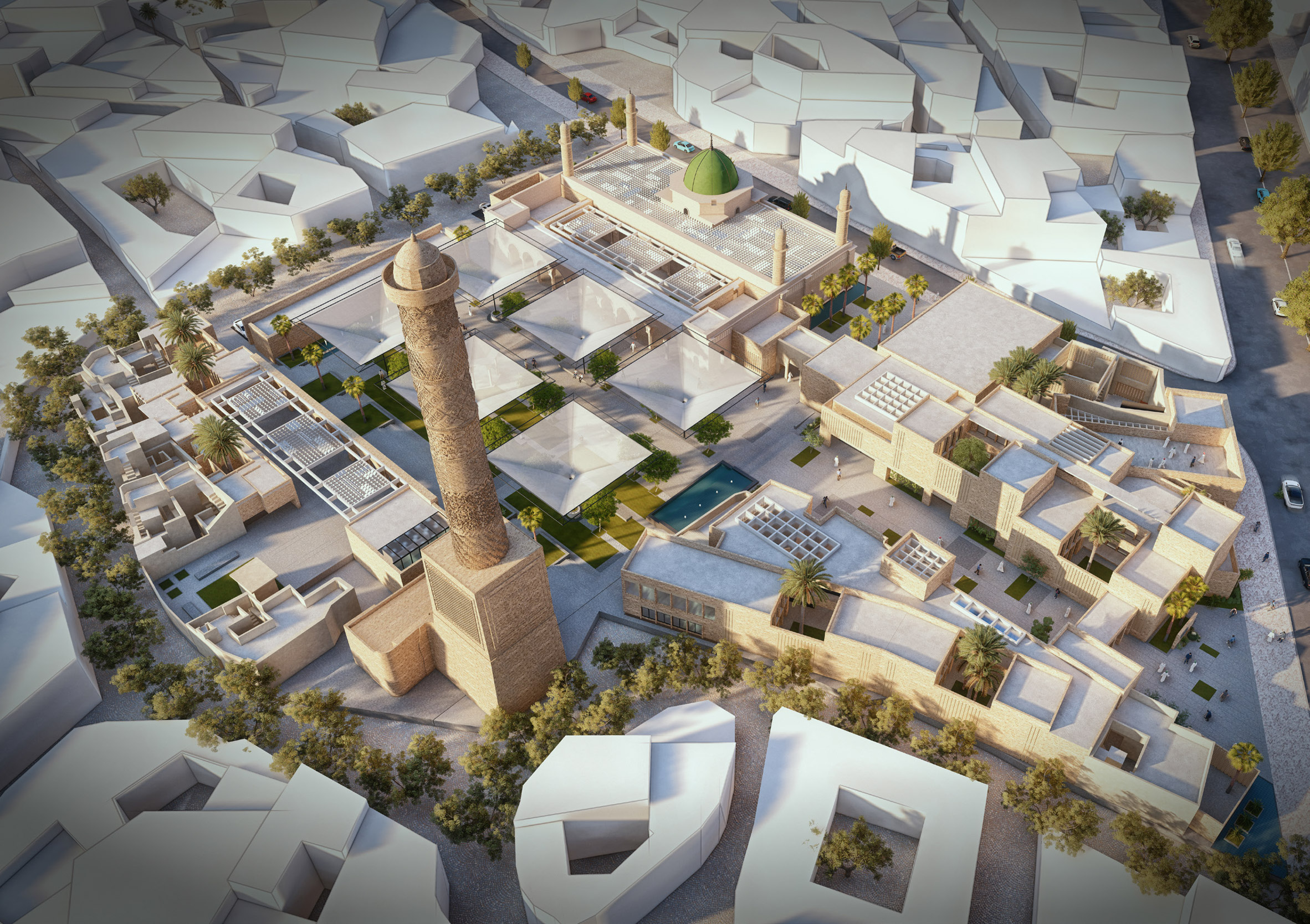This detailed aerial view captures what appears to be a meticulously crafted architectural model of a city layout. Dominated by an assortment of white buildings, the model presents various shapes including squares, ovals, and other geometric forms. Central to the display is a significant area featuring a mosque with a tall spire. Surrounding this focal point are numerous additional structures along with covered green spaces, walkways, and meticulously placed miniature trees. To the right of the layout, a road populated with car models and tiny black-and-white stick figure inhabitants adds a touch of realism. Despite the lifelike representation, the absence of textures and shading on the peripheral buildings suggests this is indeed a model or render, giving a wireframe-like appearance to the non-detailed structures. This architectural representation skillfully combines intricate details with an overarching simple design to visualize a potential city under development.